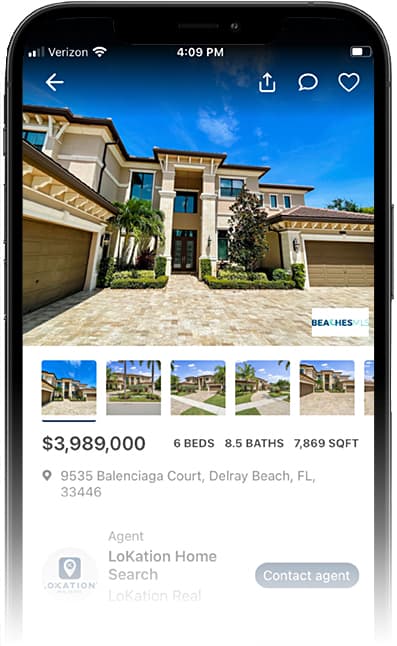The image showcases a stunning house listed on a Verizon phone, displaying the date and time as 4:09 PM with Wi-Fi enabled. The house, located at 9535 Balenciaga Court in Delray Beach, Florida, is priced at $3,989,000. It boasts 6 bedrooms, 8.5 bathrooms, and a total area of 7,869 square feet.

The property is presented with a clear blue sky and fluffy clouds in the background, complemented by meticulously maintained shrubbery. The house features a double car garage along with an additional garage. 

The listing, managed by agent Lokation Home Search, includes a prominent "Contact Agent" button for potential buyers. Below the main image, there are several thumbnail photos offering different perspectives, including views of the expansive driveway, palm trees, and more of the surrounding landscape. 

Additional features on the screen include options to like, save, and comment on the listing, enhancing user interaction with the property details.